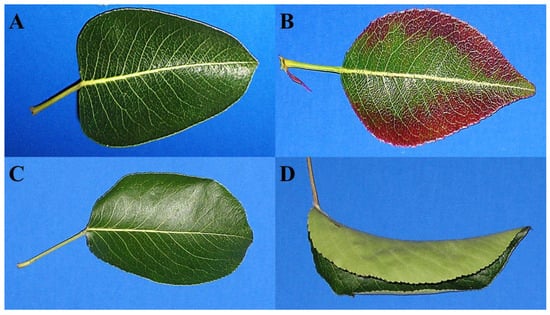The image is a collage of four distinct pictures of leaves labeled A, B, C, and D in black capital letters. Each section of the collage forms a part of a rectangular whole, with all the leaves set against blue backgrounds. 

Leaf A, located in the top left, is a healthy green leaf with yellowish veins and a triangular-round shape reminiscent of a pear. Leaf B, positioned to the right of A, has a similar shape but features red tinges along its edges, indicating the initial stages of decay. 

Leaf C in the bottom left mirrors Leaf A but appears slightly more circular and starts to fold inward, showing more pronounced curvature. Leaf D, positioned to the right of C, is significantly curled and appears dry, with a dull green coloration, suggesting it is in the final stages of deterioration.

Overall, the image captures the progressive stages of a leaf from being healthy to folding over in its final stages before dropping off.